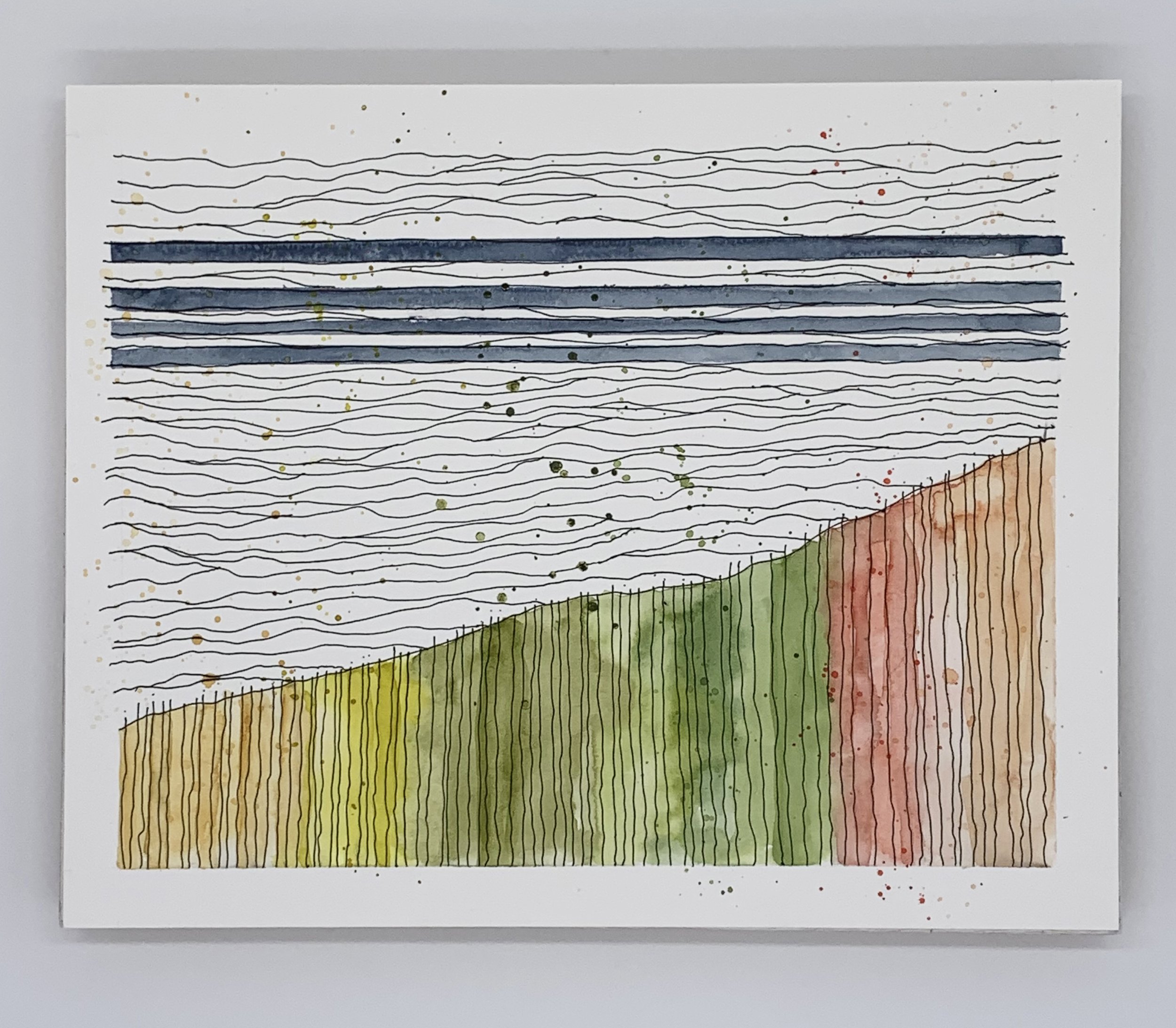The image features a single central painting, predominantly occupying the space against a grayish-white background, possibly indicative of an indoor art display or an art show. The painting itself is framed in gray and presents vertical lines that start as tan at the bottom and progressively transition to lime green, medium green, burnt orange, and finally brown, with these lines increasing in height as they ascend. Additionally, the painting is intersected by thin black lines running horizontally, coupled with five thicker black horizontal lines. The overall color palette within the image includes gray, white, black, yellow, orange, pink, and green, with the artistic nature of the piece emphasizing abstract and unstructured design elements. There is no text visible in the image.